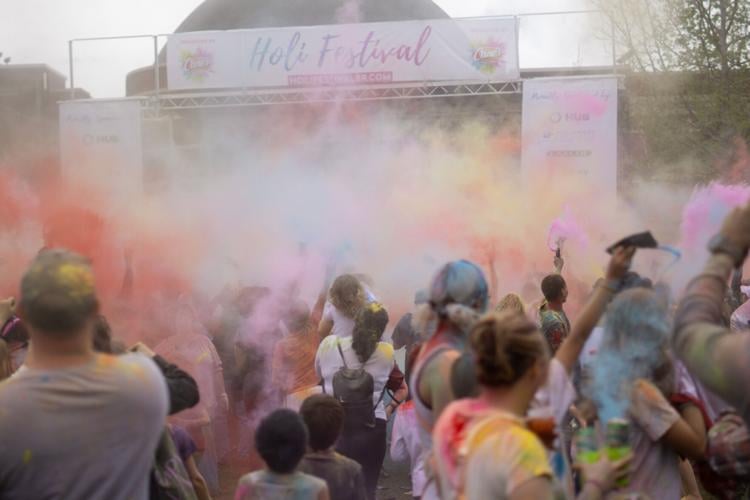This vibrant photograph captures a lively scene at the "Holi Festival," as indicated by a cursive pink and blue font banner atop a white stage with a metal frame foundation. The landscape layout image is filled with a crowd of people, primarily dressed in white shirts that are now splattered with a rainbow of colors—pink, blue, red, orange, yellow, and purple. These vivid colors permeate the air, creating a thick, colorful smoke that obscures the stage and envelops the entire area. The crowd below is a mix of children, adults, men, and women, all enjoying the festive atmosphere, reminiscent of color runs where participants are doused in vibrant powders. In the background, a few trees and a dome-like structure are vaguely visible through the haze of colors, enhancing the dynamic and joyous energy captured in this daylight scene.